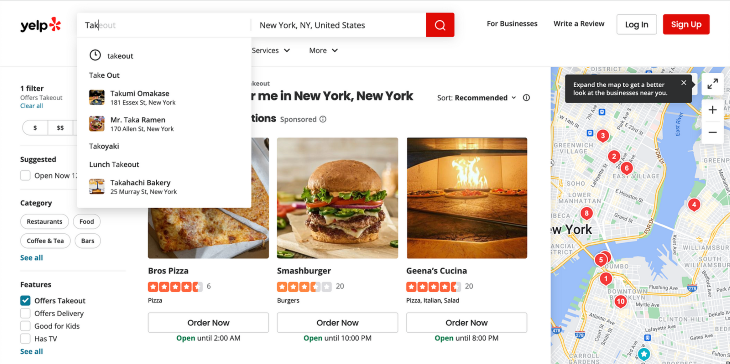The screenshot captures a Yelp search results page with several interface elements clearly visible. In the top left-hand corner is the iconic Yelp logo, a small red flower-like design, accompanied by a text box where a search query, "takeout," is being typed, though it appears unfinished. Adjacent to this is another text box indicating the location, "New York, New York, United States." Following these is a prominent red search button featuring a magnifying glass icon. Nearby, options for "For Businesses," "Write a Review," "Log In," and "Sign Up" are visible.

Beneath these, the results section displays images of various restaurants and their offerings. "Bros Pizza" is illustrated with an image of pizza, "Smashburger" shows a succulent burger, and "Greena's Cucina" features an ambiguous item baking in an oven. Each restaurant listing includes star ratings and "Order Now" buttons, along with their respective closing times like 2 AM, 10 PM, and 8 PM.

On the right side of the page, a map showcases multiple red markers pinpointing restaurant locations. The left side of the screen includes filter options such as "Offers Takeout" with an option to "Clear All," a series of dollar sign symbols to indicate price ranges, and a suggestive "Open Now" checkbox. Below these, categories like "Food," "Coffee & Tea," and a "See All" option are displayed. Further down, under "Features," checkboxes for criteria like "Offers Delivery," "Good for Kids," and "Has TV" are listed, with only "Offers Takeout" currently selected. A "See All" link is provided for additional features.